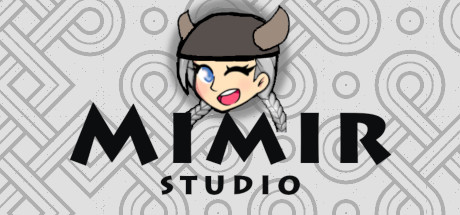Against a gray and white abstract background featuring swirls, squares, and circles, an animated cartoon of a lady Viking is prominently displayed in the center. She wears a dark brown Viking helmet adorned with lighter brown horns. Her face, drawn in flesh tones, is turned slightly sideways but she looks forward with one blue eye open and her left eye winking. Her mouth is open, revealing a pink tongue and some teeth. Her gray hair is braided, cascading down each side of her head. Below the cartoon, bold black text spells out "MIMIR Studio," taking up about a fourth of the image in height and centered beneath the drawing.